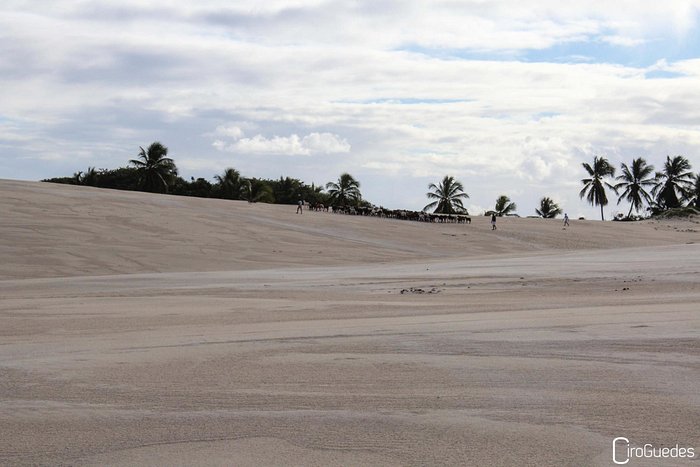This photograph captures a daytime scene at a beach devoid of water, dominated by expansive sand that shifts from a flat surface in the foreground to ascending dunes in the distance. The sand displays a range of colors from tan to light beige with touches of gray. The sky above is partly cloudy, revealing patches of blue, especially vibrant towards the top right. In the middle and far right of the image, there are three tiny, distant figures walking on the beach, appearing to herd animals, possibly cattle. Green palm trees stretch across the horizon, with clusters primarily to the right and center, their crowns the only visible parts. This scene resembles a desert oasis. In the bottom right-hand corner, the phrase “zero greetings” is faintly visible.